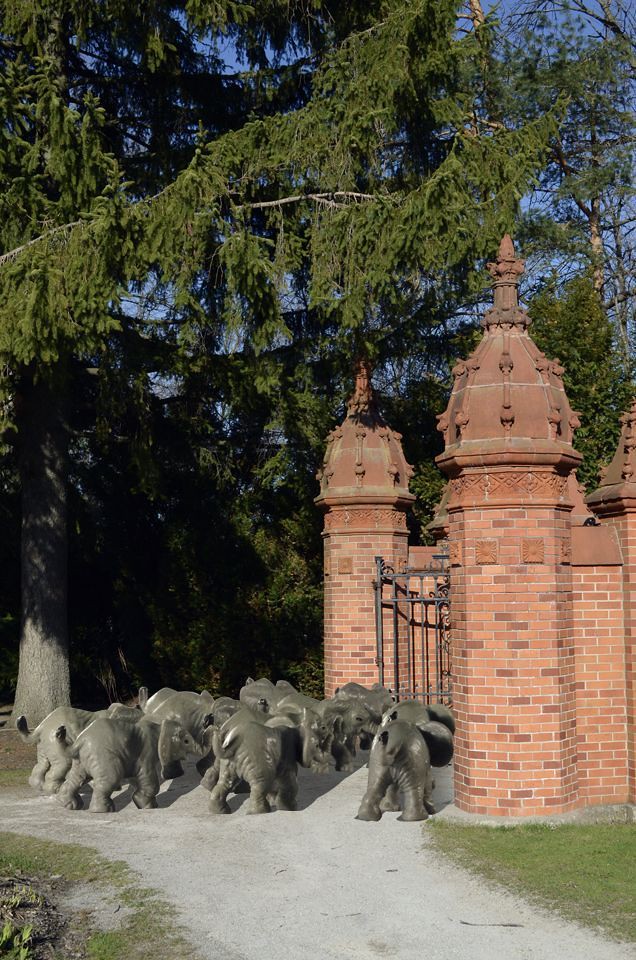This is a daytime color photograph capturing an elaborate red brick entrance to a grand house or castle. The entrance is defined by tall spires or columns capped with dome-shaped tops, adorned with crosses. A wrought iron gate, approximately six to seven feet tall, stands proudly in the middle. At the base of this gate stands a herd of small, gray elephant sculptures, resembling baby elephants, seemingly charging or walking towards the entrance. They are situated on a pathway composed of gravel and sand. To the right, there is a patch of grass, some of which appears worn out. The scene is shrouded by tall cedar trees with green, dangly branches casting shadows over their trunks and to the left side of the image. The sky is bright blue, indicating a sunny day, yet no people or vehicles are present. The photo offers a clear view of the elaborate, panel-like tops of the brick columns and the serene natural surroundings.